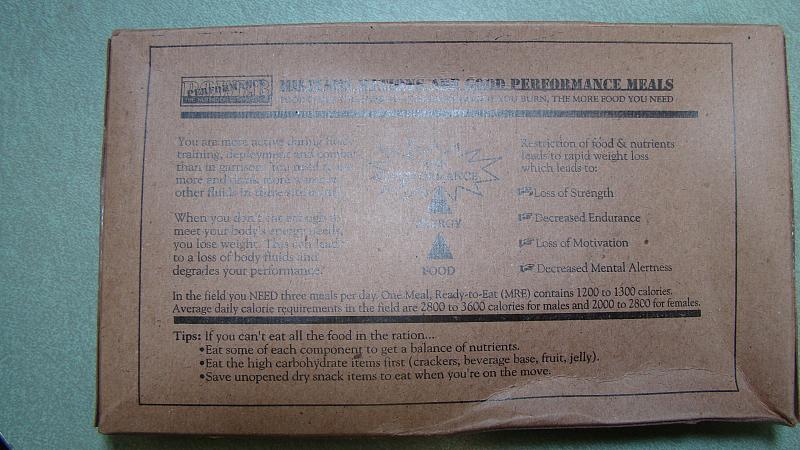This image fills the entire horizontal frame and features a piece of cardboard with a black border and black text in the middle, set against a grayish-blue background. The piece of cardboard has light reflecting off the center, obscuring some of the text. At the top right, "Performance Meals" is legible. Below it, on the right side, there's a partially readable line that states, "burn, the more food you need," while the left side is not visible.

In the middle of the cardboard, there are several drawings surrounded by text on either side. The drawings include a starburst, something indistinguishable beneath it, and a pyramid with the word "food" underneath. 

At the bottom, clear instructions and tips are written:
- "Tips: If you can't eat all the food in the ration,"
- "Eat some of each component to get a balance of nutrients."
- "Eat the high carbohydrate items first: crackers, beverage base, fruit, jelly."
- "Save unopened dry snack items to eat when you're on the move."

All the text on the piece of cardboard is rendered in black.